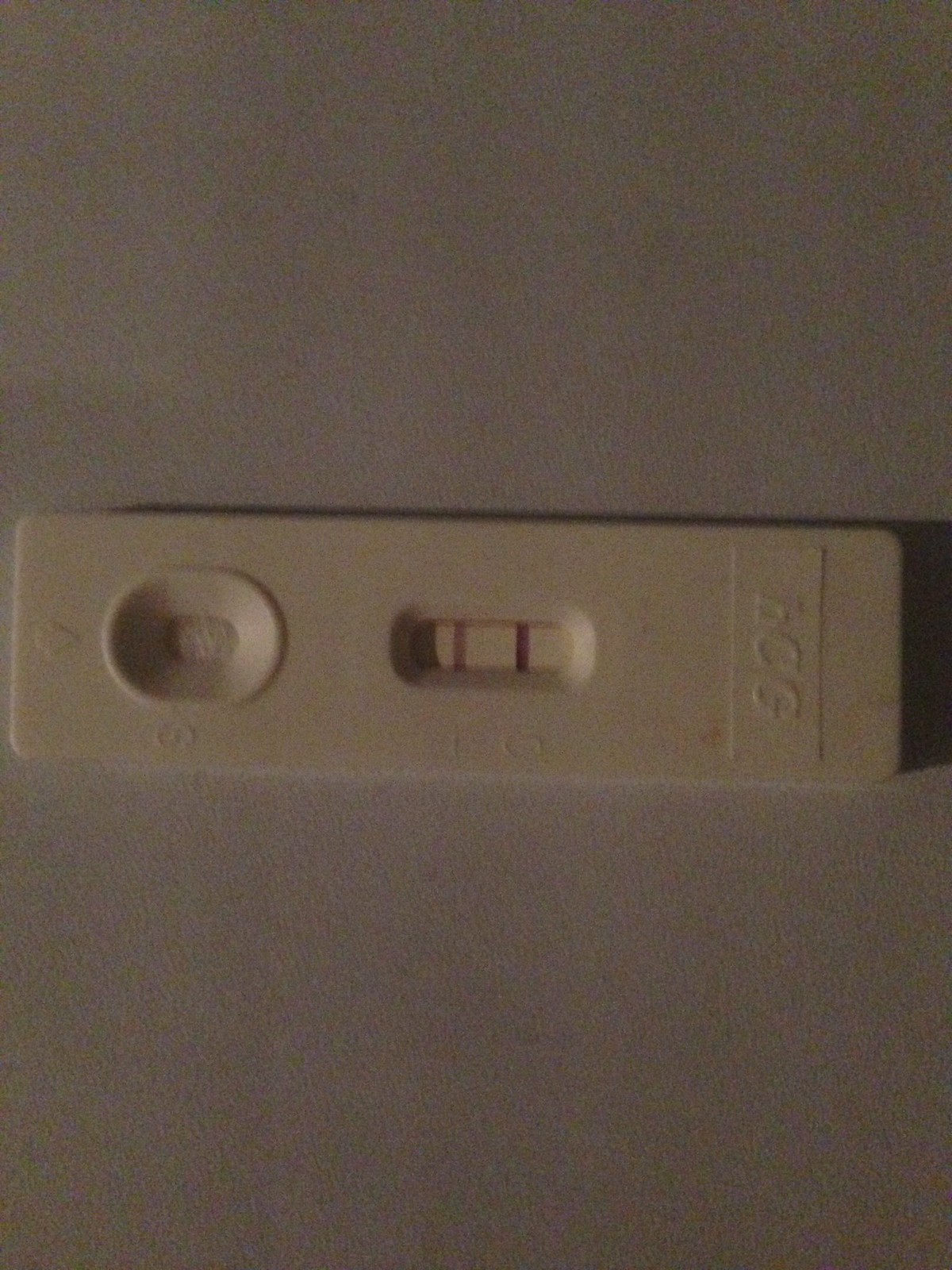This image depicts a slightly out-of-focus, vertical rectangular photograph featuring a flat piece of molded plastic prominently placed at the center. The plastic piece, characterized by its elongated, narrow shape and horizontal alignment, is white. Centrally embedded within this plastic piece is a small, horizontal glass tube with a leveling bubble, typical of those found in leveling rulers. Adjacent to the tube, two vertical red lines serve as reference markers. On the left, the plastic displays an arrow cut into its surface, pointing to a bowl-shaped indentation with a central hole, providing a functional yet unidentified purpose as denoted by the adjacent letter 'S' and a short line marking the indentation. The right side of the plastic has three letters, "HCG," embossed vertically along its edge. The backdrop of the image is a muted dark white wall, providing a neutral contrast to the plastic component.